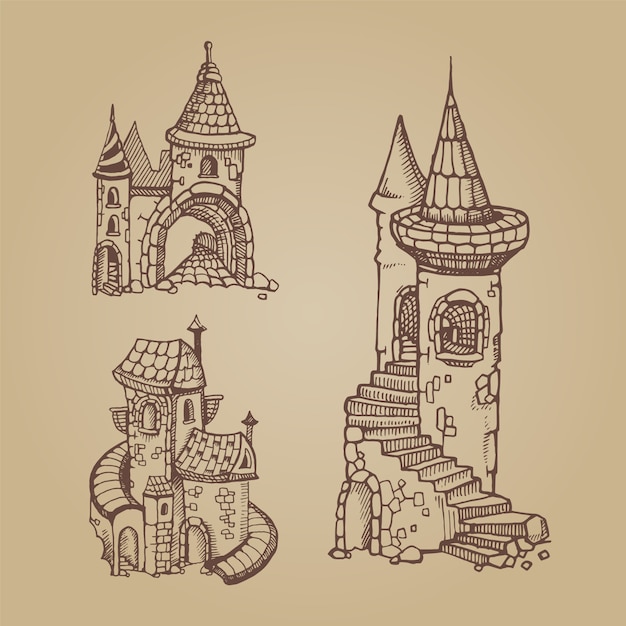This detailed illustration, crafted with brown ink on light brown paper, depicts three distinct architectural designs. On the left side, the uppermost image features a grand building highlighted by a prominent tower capped with a conical roof. Adjacent to this is a smaller tower positioned to its left, complete with an open archway that provides a view into a tunnel-like structure at the front of the building.

Directly below, the second illustration reveals a two-story building adorned with dual chimneys. A winding staircase commences at the bottom right, elegantly curving around to the left, leading to an arched doorway that offers a glimpse of stairs within.

Dominating the right side, the largest image showcases an impressive tall tower, topped with a conical roof, accompanied by a secondary tower situated behind it. An arched doorway is positioned at the bottom left, and a grand staircase spirals around the building, seamlessly integrating into the architecture of the second tower. The cohesive use of ink and paper tones enhances the detailed intricacy of these architectural depictions.